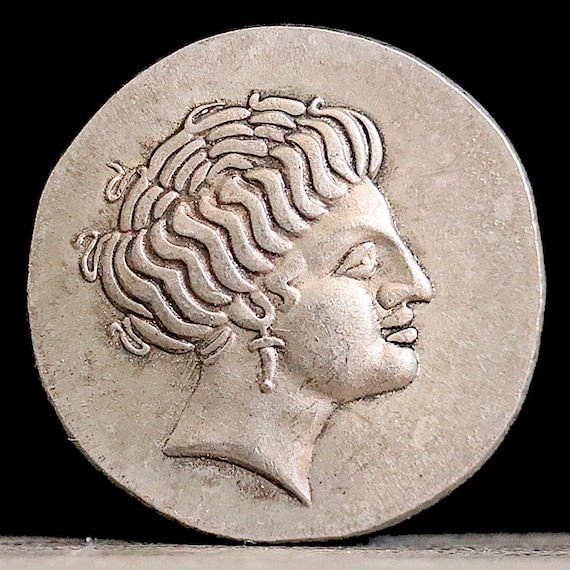This high-resolution photograph showcases an ancient silver coin, likely of Greek or Roman origin, captured in professional lighting against a stark black background. The coin, displayed upright and resting on a thin, barely noticeable cloth at the bottom, features the intricate profile of a figure with distinctly European features, characterized by a prominent Roman nose and coily hair that evokes the mythological Medusa, giving the illusion of serpents. The finely detailed bust, facing right, includes a long, dangly earring, with the figure’s wavy hair, slightly open mouth, and forward-gazing eyes, all carved in relief. The image, possibly part of a museum collection, effectively highlights the coin's historical significance and craftsmanship.